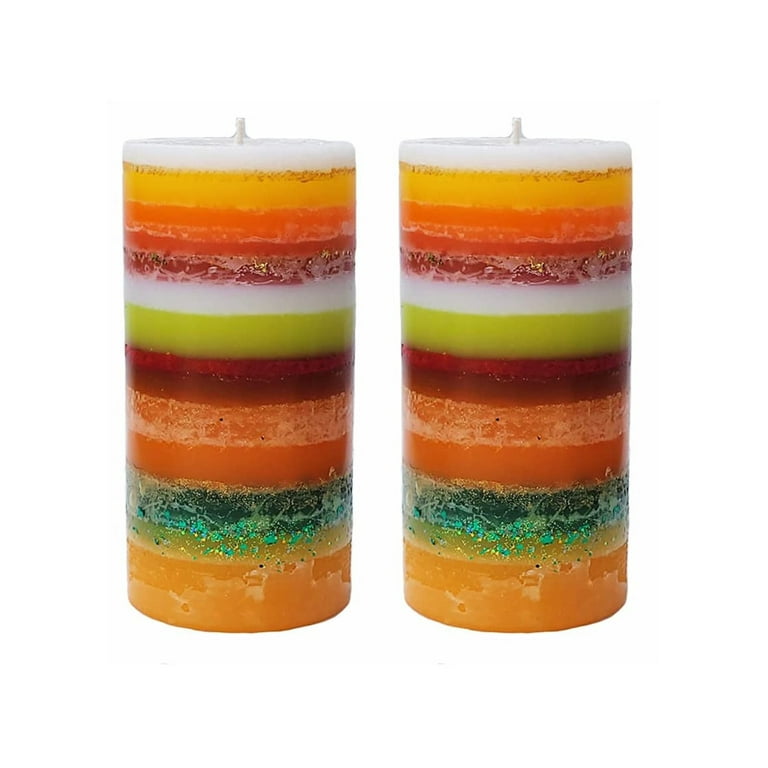This color photograph features two identical wide pillar candles, each composed of multiple colorful layers, standing side by side against a plain white background. Starting from the top, the candles exhibit a white wick followed by consecutive layers of white, yellow, lighter orange, darker orange, and almost red, eventually transitioning to brown, white again, then green, then a deep red, then a mix of orange and white, another orange layer, concluding with green and lighter orange at the bottom. These decorative candles appear unused and could serve as perfect Thanksgiving decor. Their vibrant and varied hues, with elements of glittery gold green interspersed, enhance their festive and appealing aesthetic, making them suitable for a sale display as well.